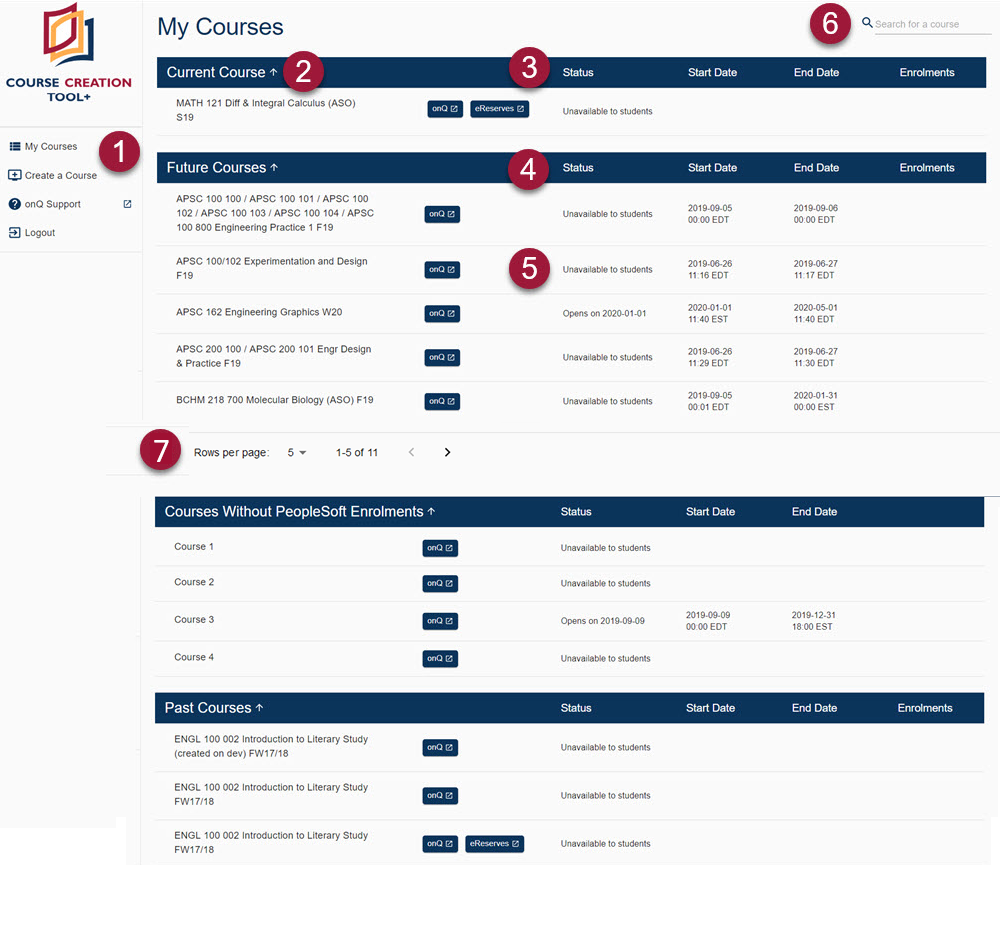Certainly! Here's a cleaned-up and detailed caption:

---

**Screenshot of an Online Course Creation Tool Interface**

This square-format, color screenshot captures the interface of an online course creation tool, akin to platforms like Coursera. The interface is dominated by hues of dark blue and dark red, with a distinctive logo featuring three interconnected, window-like icons in dark red, orange, and dark blue – a visually appealing element that stands out.

The interface reveals four main navigation tabs located on the left side: "My Courses," "Create a Course," "ONQ Support," and "Log Out." The user in the screenshot has selected the "My Courses" tab, unveiling several sections related to course management. 

The currently active section lists a math course titled "Math 101: Differential and Integral Calculus." This course is marked as "unavailable to students" and lacks specific start and end dates. Below this section, there are listings for future courses, emphasizing subjects within the scientific domain such as "Experimentation Design," "Engineering Graphics," and "Molecular Biology." Each of these listings includes their status updates along with their respective start and end dates.

The organized presentation and detailed options indicate a robust platform meant for managing and creating academic courses, providing users with essential tools to facilitate online learning.

---